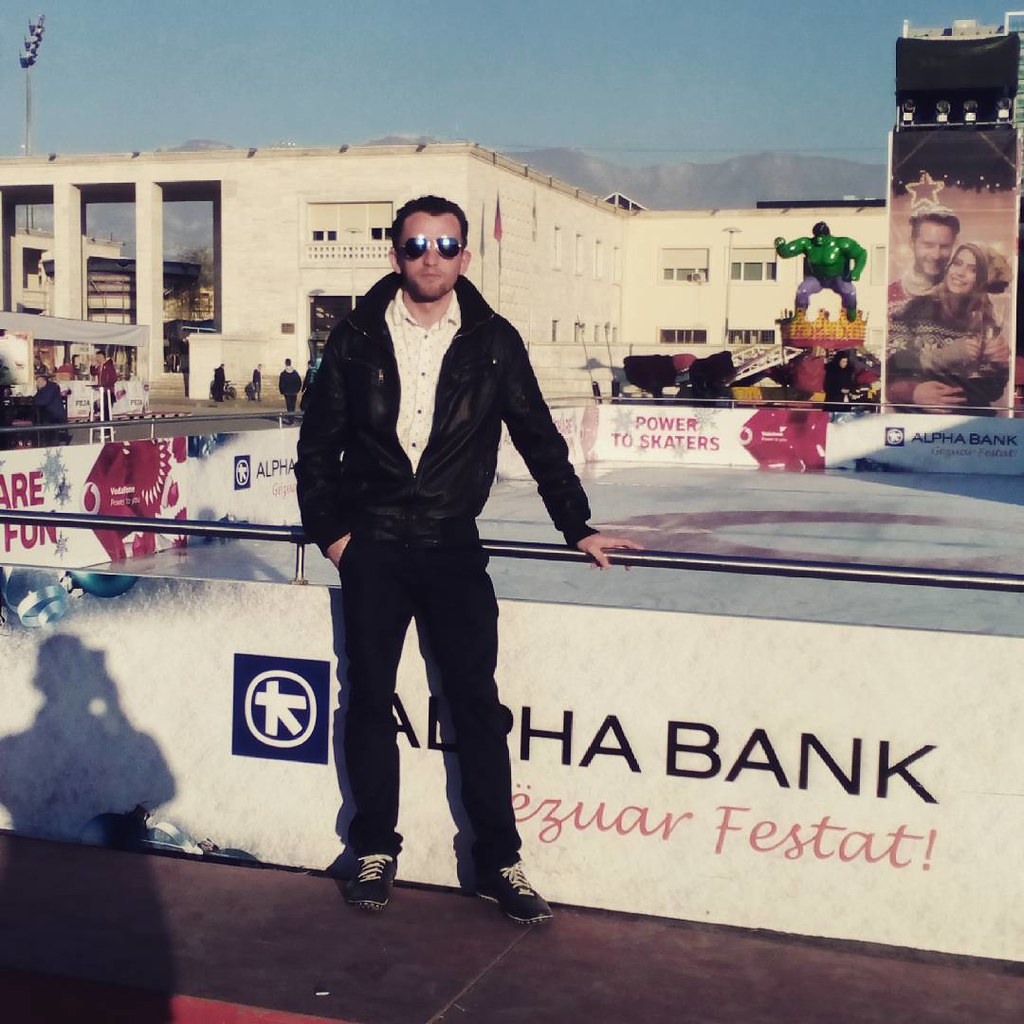In this outdoor photo, a man with short hair and a goatee is casually posing, leaning on a black railing with his left hand while his right hand is in his pocket. He is sporting a black leather jacket over a white undershirt, jeans, black tennis shoes, and dark aviator sunglasses. The scene appears to be in front of a skating rink, likely indicated by the icy surface and the tagline "Power to Skaters" on a nearby sign. Prominently behind him, there's a large white sign for "Alpha Bank" in black text, with a foreign word in light red cursive underneath. In the background, there's a big white concrete building with windows and a vibrant statue of the Incredible Hulk, vividly green with black hair and purple pants, standing atop a red and yellow crown. The uppermost part of the image reveals a blue sky and distant mountains. Additionally, there are banners around the rink, one showing a man and a woman embracing beneath a star, while advertisements adorn the railing. The shadow of the person taking the picture is visible in the bottom left corner.